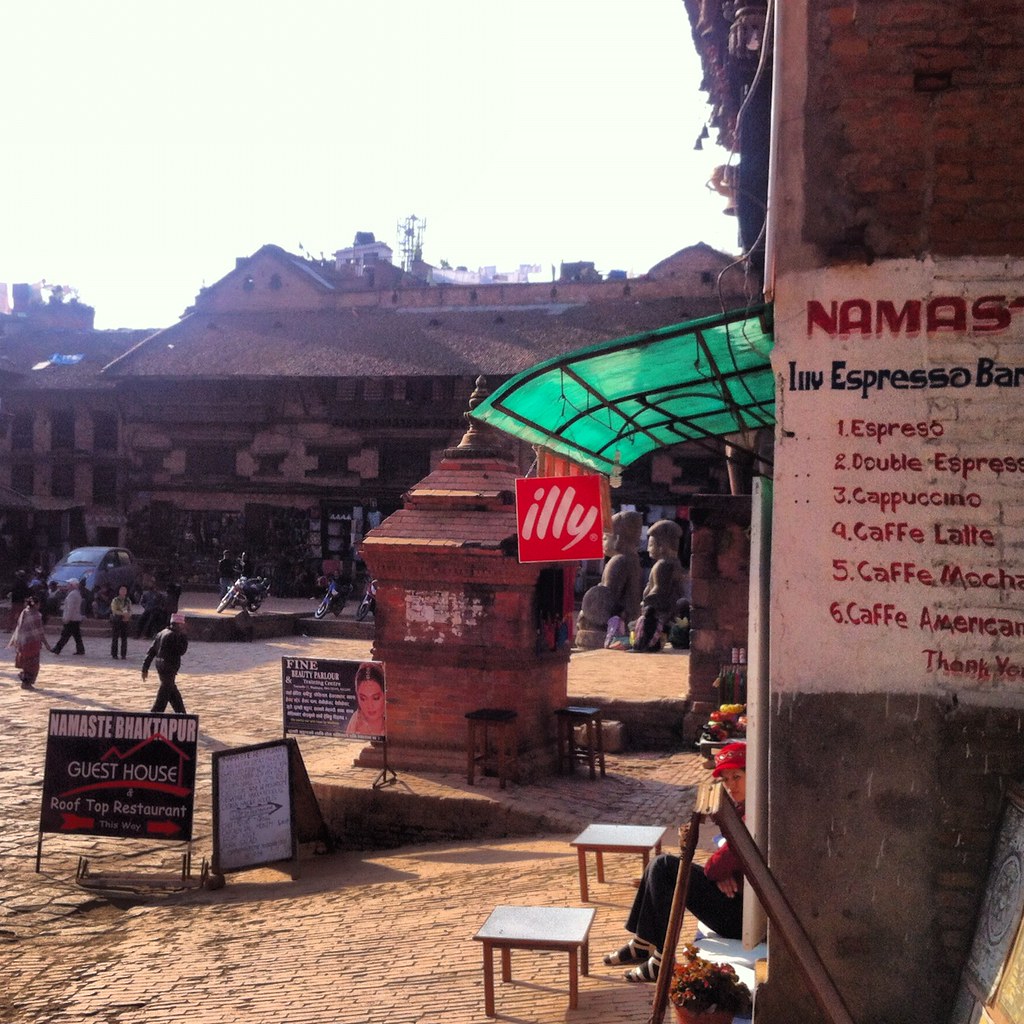This detailed image shows a vibrant street scene in a small town, possibly in India, with a bright sunny sky that appears almost white. The foreground prominently features a painted sign on a concrete wall listing a menu for "Namaste, INV Espresso Bar," offering one espresso, two double espresso, three cappuccino, four caffe latte, five caffe mocha latte, and six caffe americana, with a 'Thank you' note. Adjacent to this, there's a green awning with a red square Illy coffee logo. 

Below the awning, a person wearing dark pants and a red cap is seated at a small table outside the coffee shop, next to a sandwich board sign advertising "Namaste Bank Thapur Guest House, Rooftop Restaurant." This board displays red and white designs, including an arced line and a triangular lightning bolt.

In the background, a shingle-roofed building with multiple peaks houses various other establishments, marked by additional signs, one of which includes a picture of a woman. The bustling street features a mix of brick sidewalks and larger roadblocks, with several people and a light-colored car with a curved back end navigating the area. Notable individuals captured include a person in a white cap with a white shirt and dark pants, a woman in a plaid skirt and white top, and a man dressed in black walking forward.

To the right edge of the scene, another section of the menu can be seen with a partially obscured sign in red and black lettering. Various small statues and additional signs litter the street, adding to the lively, slightly chaotic atmosphere of this historic town.